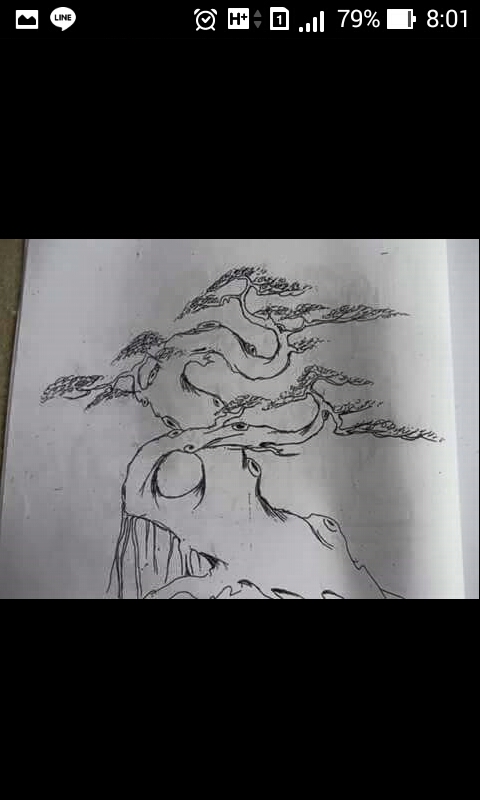Screenshot Details:  
- **Notifications:** The top of the image features several notifications, including an alarm clock icon, a network connection indicator showing impressive speed, a battery indicator at 79%, and the current time reading 8:01. There is also a notification specific to the screenshot we are viewing and a message from Line Messenger.
- **Background:** The backdrop of the phone screen is set to black, giving the overall image a stark contrast.
- **Main Image Description:** The primary focus of the screenshot is a striking black-and-white illustration of a tree with elements that suggest Japanese or Chinese artistic influence. While reminiscent of a bonsai tree, this depiction is much larger and more intricate. The tree's design features multiple large trunks that twist and intertwine in a fluid, almost dance-like fashion, rather than straight vertical growth. Around the center, these trunks form a circular shape, adding to the aesthetic complexity. Smaller branches sprout from these main trunks, following the same intertwined and curved pattern. Notably, there are visible stubs where branches either broke off or were pruned, further adding to the tree's character. The roots of the tree are depicted extending into the ground, anchoring the entire composition firmly within the black and white medium. The fine detail captures the organic interlacing and natural elegance of this tree, making it a captivating piece of artwork within the digital screenshot.